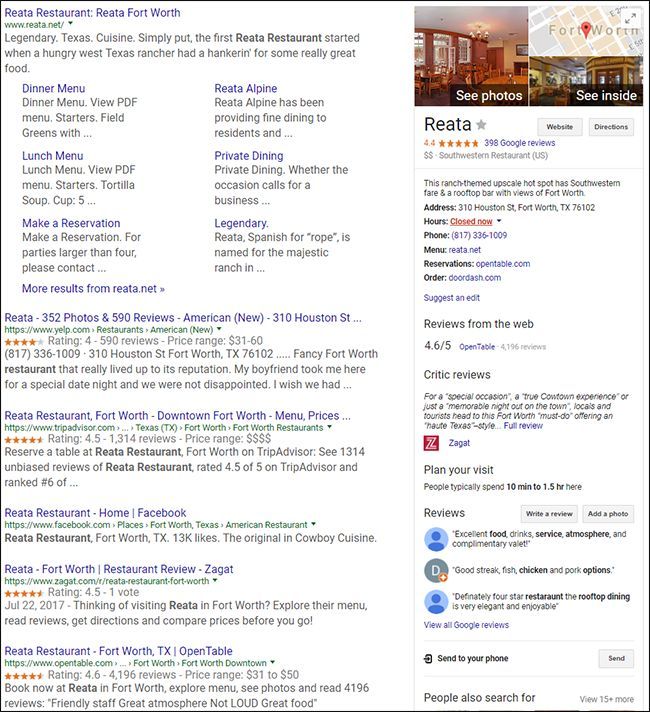In this image, we are presented with a screenshot of a Google search results page for Retta Restaurant in Fort Worth, Texas. On the left side of the screen, several link addresses are displayed in sequence. The top link reads "Retta Restaurant, Retta Fort Worth" followed by "Retta 352 Photos and 590 Reviews, American New." Below these, we find links to "Retta Restaurant, Fort Worth, Downtown Fort Worth, Menu Prices," "Retta Restaurant, Home, Facebook," "Retta Fort Worth Restaurant Review, Sackett," and finally "Retta Restaurant, Fort Worth, Texas, Open Table."

On the right side, the screenshot showcases images from the restaurant alongside a small map indicating the location. The listing highlights that Retta has a rating of 4.4 stars based on 398 Google reviews. It describes the restaurant as a ranch-themed, upscale hotspot featuring a southwestern flair and a rooftop bar with views of Fort Worth. The section provides essential details such as the address, hours of operation, phone number, menu options, and reservation links. At the bottom right corner, reviews are visible, offering further insights into patrons' experiences at Retta.